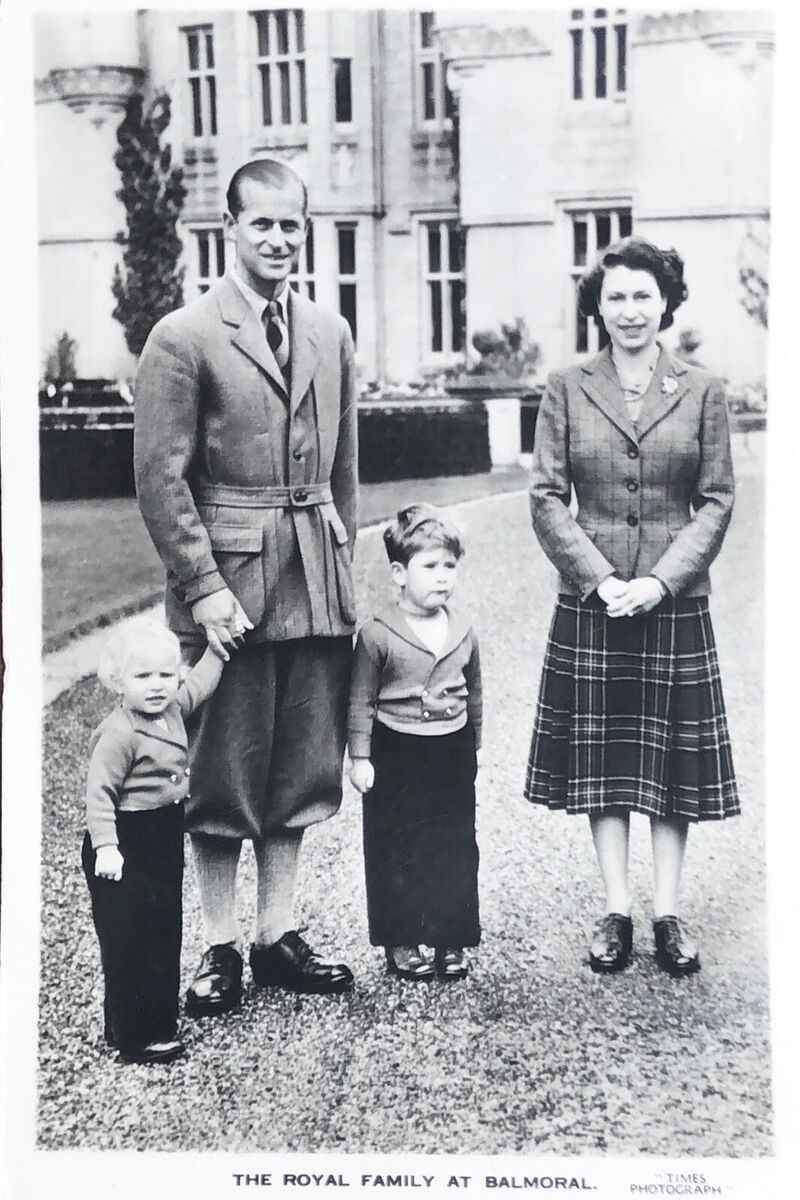This black-and-white photograph, captioned "The Royal Family at Balmoral" at the bottom, and marked as a Times photograph, captures a youthful Queen Elizabeth II on the right-hand side, dressed in a plaid blazer and matching skirt. To her left is her husband, Prince Philip, attired in a jacket with a belted waist, poofy knee-length pants, likely tights, and loafers. He holds the hand of a small, brown-haired child wearing a sweater and a skirt, while another young girl, identified by her white hair and dressed in a sweater and black pants, stands to his left. The family is positioned in front of the stately and historic Balmoral Castle, all looking directly at the camera with the Queen's hands gently clasped in front of her. This image, likely from around 40 to 50 years ago, encapsulates a moment in time of royal family life at their private residence.